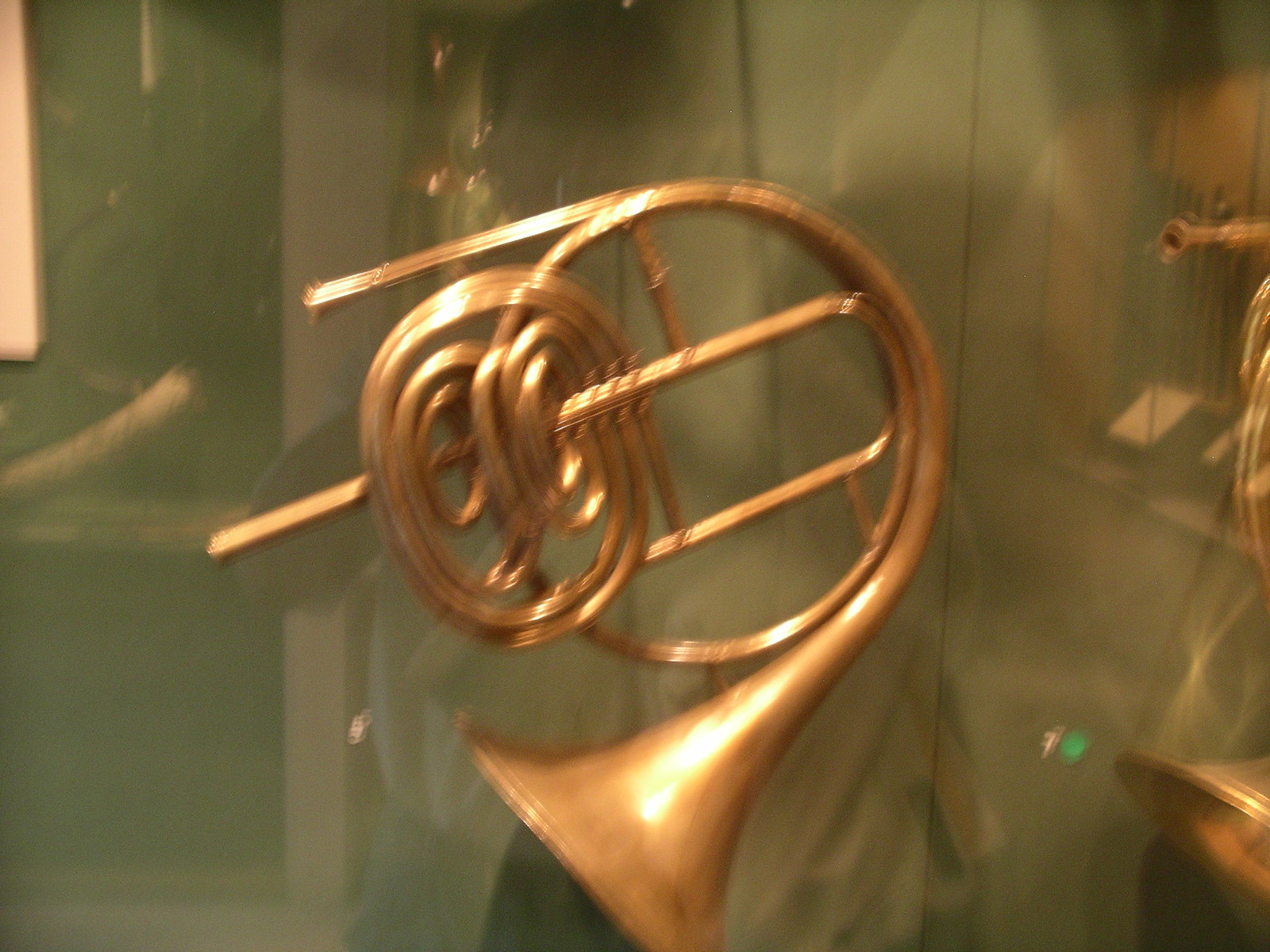The photograph captures a detailed view of a large, intricate brass wind instrument, possibly an antique horn. Its copper-brown surface is accentuated with light reflections, giving it spots of white highlights. The instrument features an elaborate design with numerous curls and circles, almost appearing knotted, suggesting it might be more decorative than functional. Positioned behind glass, the image reveals a slight reflection, adding depth and a mirrored effect to the scene. The backdrop includes an olive greenish hue to the left, and just barely visible is another similar wind instrument situated to the right, indicating a display or collection. This ornate horn, facing downward and to the left, showcases two distinct parts for blowing, hinting at its capability to produce a wide range of notes, further emphasizing its artistic and possibly historical significance.